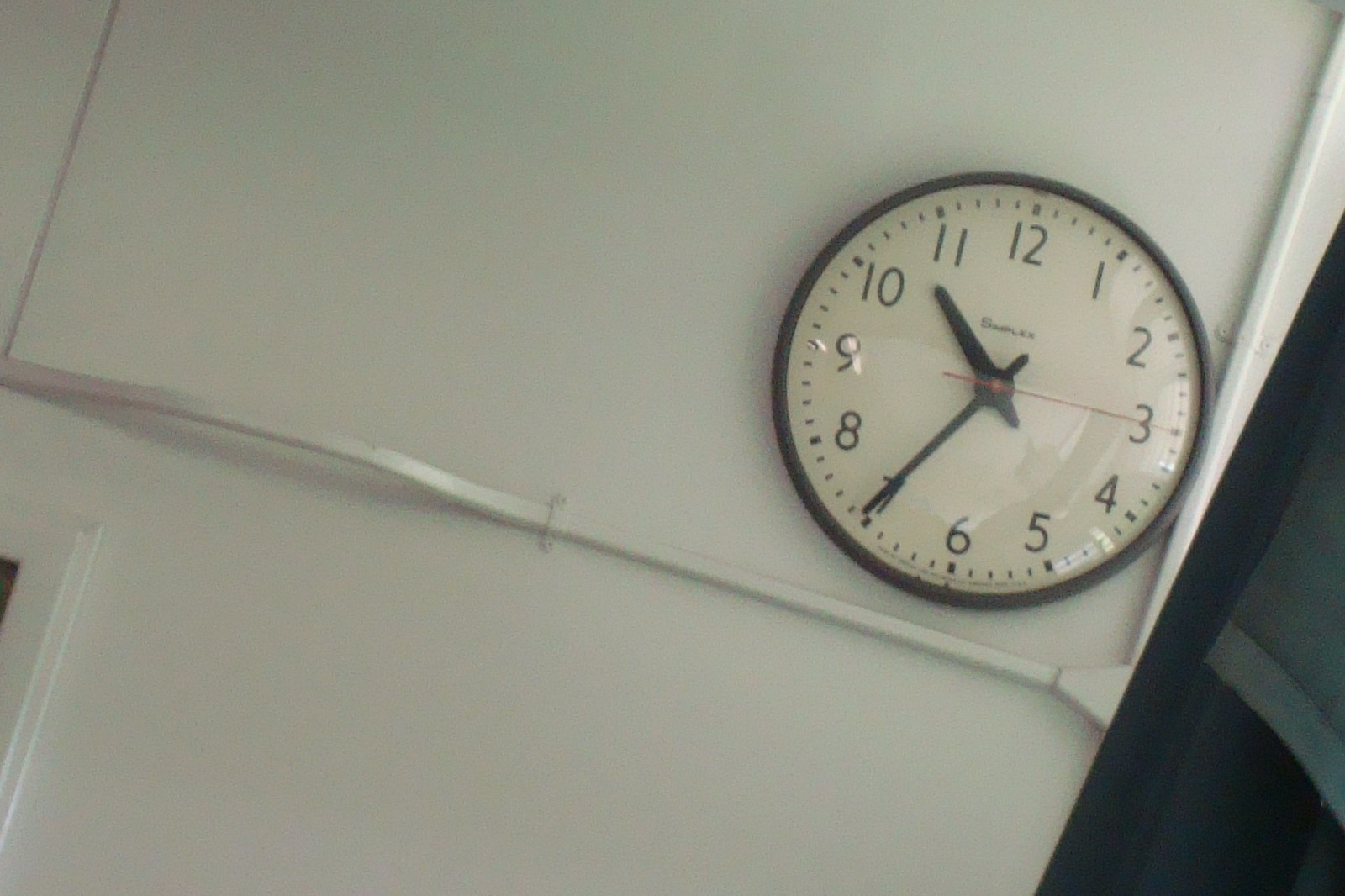This image features a minimalist clock mounted on a stark white wall, positioned near the top right corner. The clock itself has a sleek black border encasing a white face, with black numerals indicating the hours. The design is straightforward yet bold, highlighted by thick black hour and minute hands, contrasted by a slender red second hand. In the scene's periphery, the bottom left corner reveals part of a frame—likely belonging to a door or window. Meanwhile, the bottom right corner shows a piece of dark fabric, possibly a navy blue or black curtain. The simplicity of the white wall accentuates the clock's precision and the subtle elements around it.